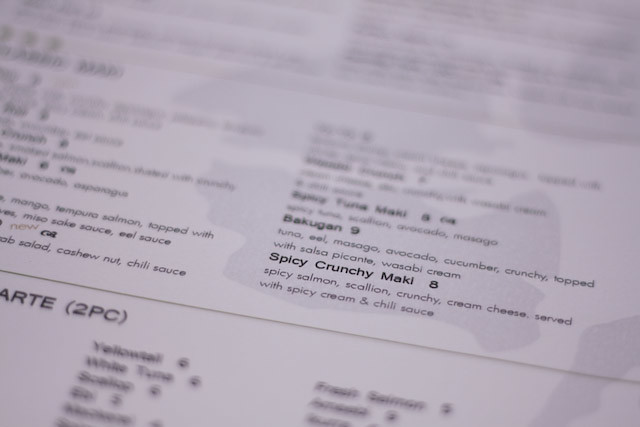The image is a close-up photograph of a restaurant menu, likely featuring sushi. The focal point of the image is a small, readable portion of the menu, which lists an item called "Spicy Crunchy Maki" priced at 8. This dish is described as containing spicy salmon, scallion, crunchy cream cheese, served with spicy cream and chili sauce. The menu itself is predominantly white with black text arranged in two columns, though the photograph is so heavily blurred that most of the writing is unreadable except for the pinpointed area in focus. Just above the Spicy Crunchy Maki, there seems to be another item that possibly reads "Bakugan," which includes ingredients like tuna, eel, masago, avocado, cucumber, crunchy elements, and is topped with salsa picante and wasabi cream. The rest of the menu text is too indistinct to decipher, and the overall image has abstract shapes and color splotches in the background.